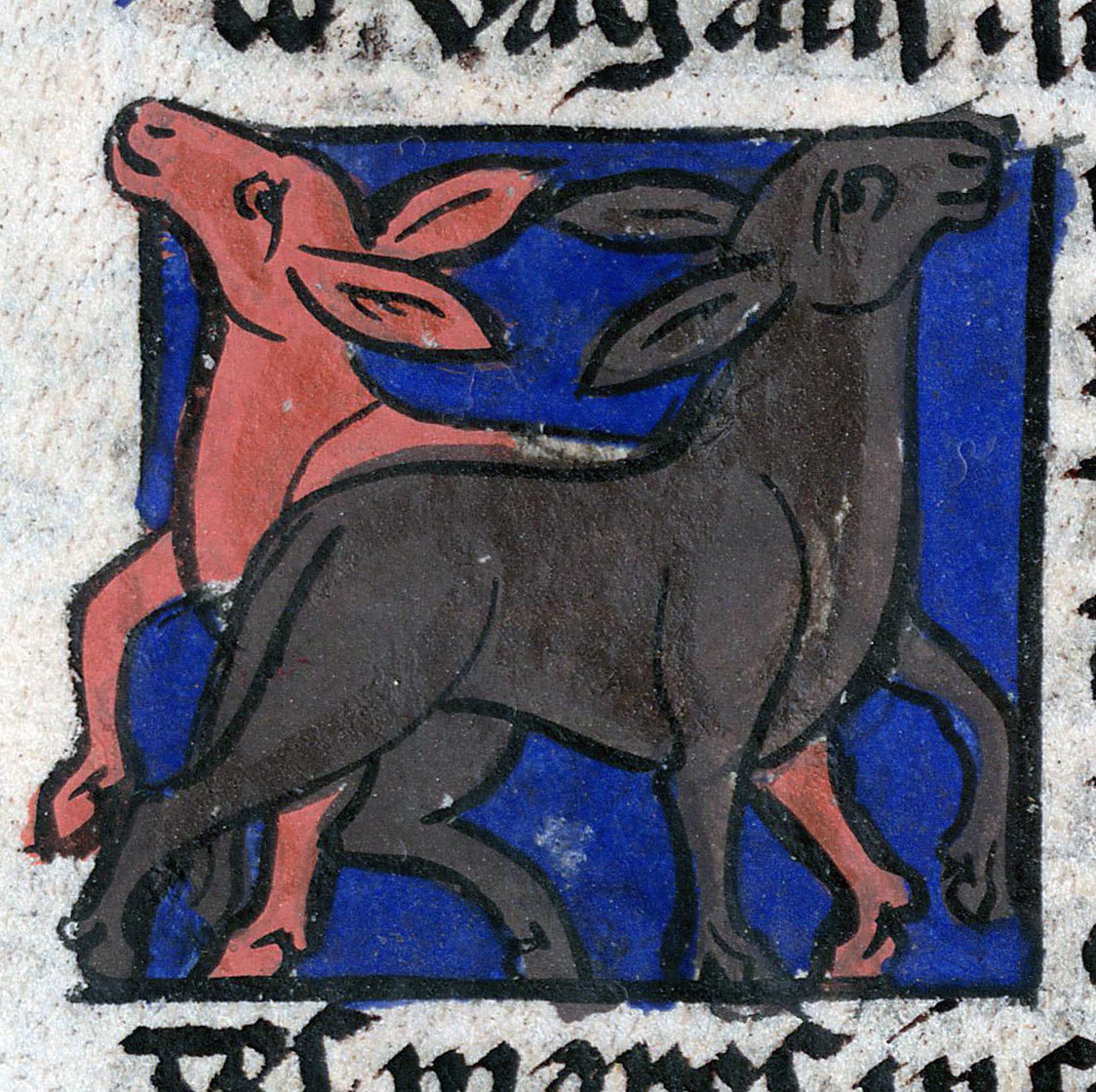This image appears to be a detailed colored drawing, possibly an excerpt from a larger piece of art. It features a simple yet striking depiction of two donkey-like animals, outlined in thick black lines against a vibrant sapphire blue square that is also bordered in thick black. The bright blue background contrasts sharply with the modeled white surface that could be low-quality paper, fabric, or marble.

The animals are presented in a cartoonish style, both with long snouts and pointy ears, their heads held high. The donkey in the foreground, facing right, is colored a very dark gray or brown. Behind it, the second donkey, facing left, is a pinkish or pale red color. The entire scene is framed by lines of black Latin text at the top, bottom, and right-hand side of the image, though these are incomplete and cut off by the frame, suggesting the image is part of a larger composition.